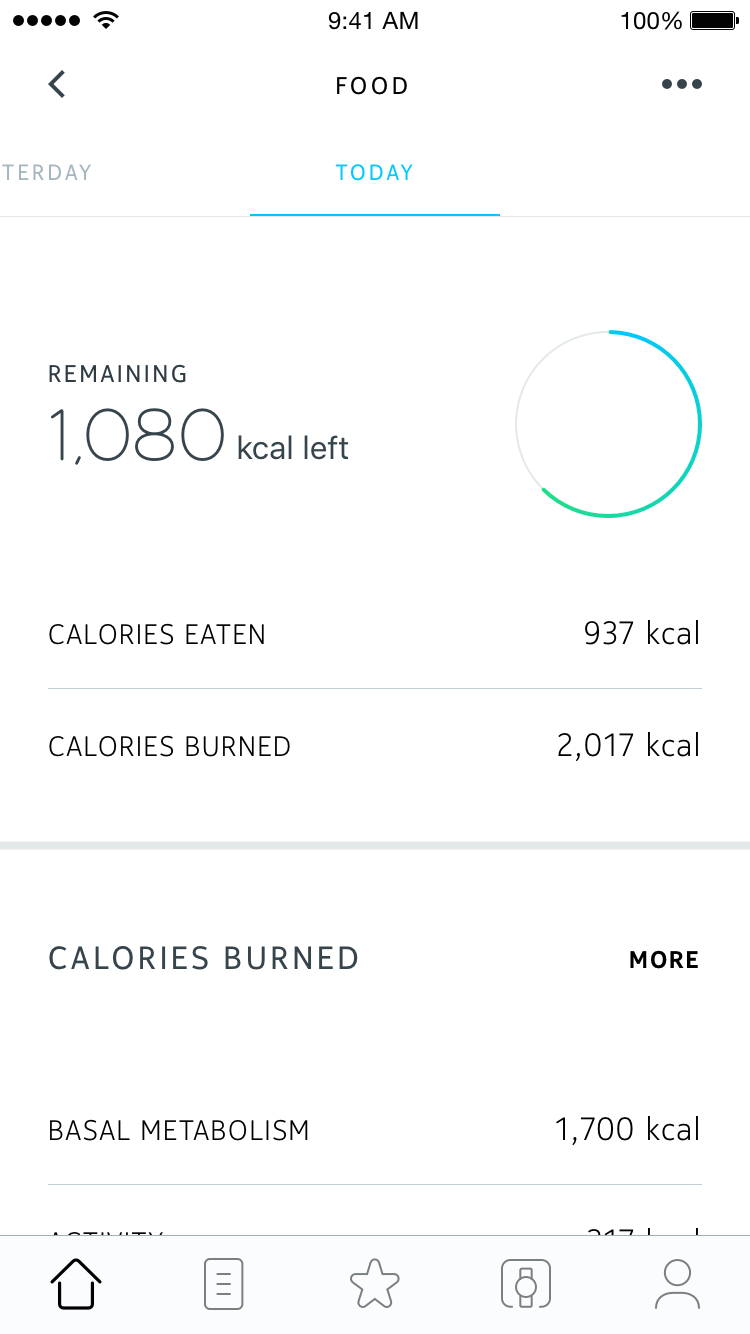A detailed screenshot of a diet and fitness app displayed on a smartphone. In the upper left-hand corner of the screen, the Wi-Fi signal icon is visible, indicating connectivity. At the very top center, the current time is shown as 9:41 AM. To the right of the time, the battery icon indicates a fully charged battery at 100%. 

The app interface is divided into various sections, with the 'Today' tab selected under the 'Food' menu. Prominently displayed in the 'Today' section, the word "Remaining" appears, showing the remaining calorie allowance for the day, which is 1,080 kcal. Below this, the calories consumed so far are listed as 937 kcal. 

Further down, there's another section titled "Calories Burned," which lists the total calories burned as 2,017 kcal. To the right of this section is a "More" option, suggesting additional information can be accessed. At the bottom of the display, there's a segment labeled "Base Metabolism," showing a value of 1,700 kcal to the right.